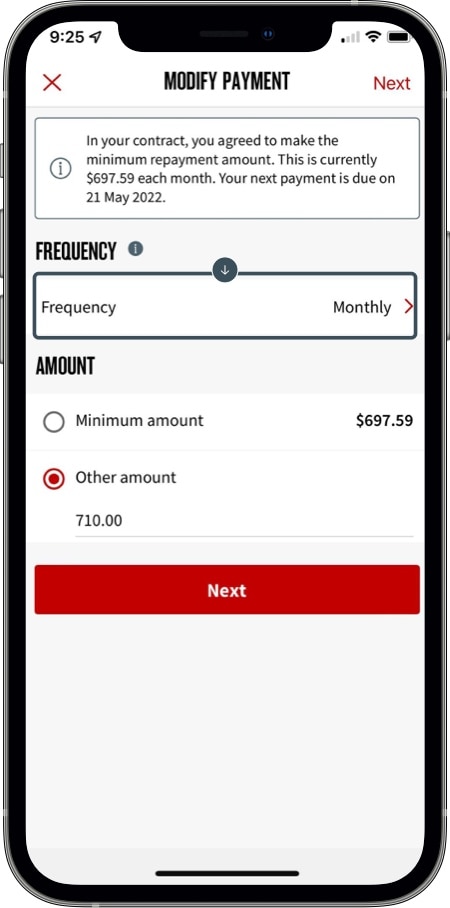The image captures a smartphone displaying a payment modification page with a predominantly white background and black text. At the top of the screen, the heading "Modify Payment" is prominently shown, accompanied by a red "Next" button on the top right. Below the header, there is a paragraph stating, "In your contract, you agreed to make the minimum repayment amount. This is currently $697.59 each month. Your next payment is due on May 21, 2022." The section beneath this text is labeled "Frequency" with "Monthly" selected and highlighted on the right.

Further down, the "Amount" section lists two options: "Minimum Amount: $697.59" and "Add Amount: $710.00." The "Add Amount" option is selected, indicated by a red checkbox next to it. At the very bottom of the screen, a prominent red button with white text reads "Next" to proceed to the next page. Lastly, on the top left corner, an "X" in red can be seen, providing an option to close the current page.